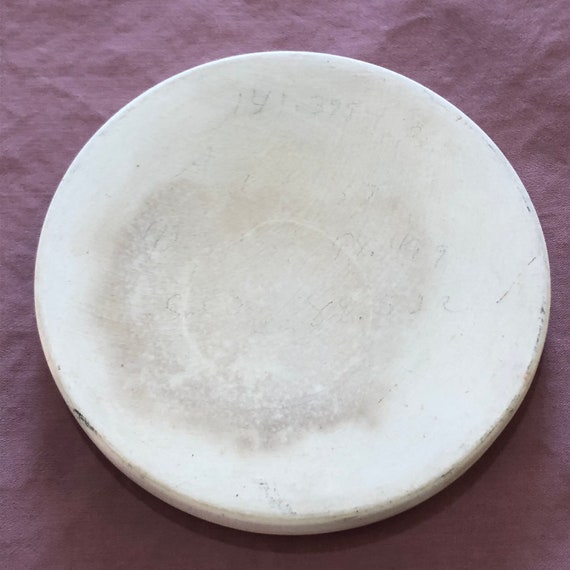The image shows an overhead view of a heavily worn white saucer or faded-out frisbee lying on a maroon or purple cloth covering a tabletop. The saucer features numerous dark, grayish ash-like markings, particularly concentrated at the center, and smudges surrounding almost all its edges, particularly accentuating wear and tear. There are faint, partially legible numbers inscribed inside the saucer, possibly reading "141371" or "14437". The saucer has a slightly curved surface with a soft indentation rather than being entirely flat. Its edges are significantly dinged and scratched, revealing a metallic undertone beneath the white coloring. The time of day appears to be daylight due to a faint light casting a soft shadow of the saucer onto the cloth below.